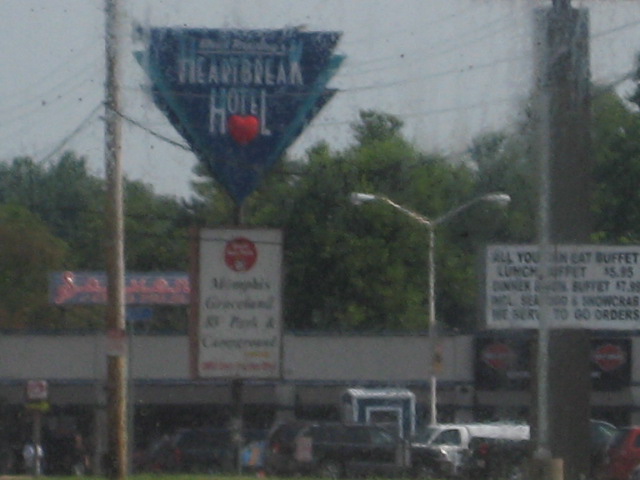The image showcases a nostalgic scene set in front of a hotel, evoking a 1940s-1950s Route 66 aesthetic. Dominating the foreground is a triangular blue sign, displaying "Heartbreak Hotel" in bold white letters, with a vibrant red heart just below the word "hotel." This sign sits above a retro-styled rectangular white sign, which bears the slightly blurred name "Memphis" and features a red circle. Surrounding this centerpiece are several parked cars spread across a spacious parking lot. A low, white-ish building stands adjacent to the lot, contributing to the vintage ambiance. 

On the right-hand side of the image, a brown pole supports a white sign advertising an "All-You-Can-Eat Buffet," accompanied by more indiscernible text. The background is rich with lush green trees, while a tall brown telephone pole rises on the left, adorned with telephone wires stretching towards a grayish sky above, enhancing the timeless feel of the scene.